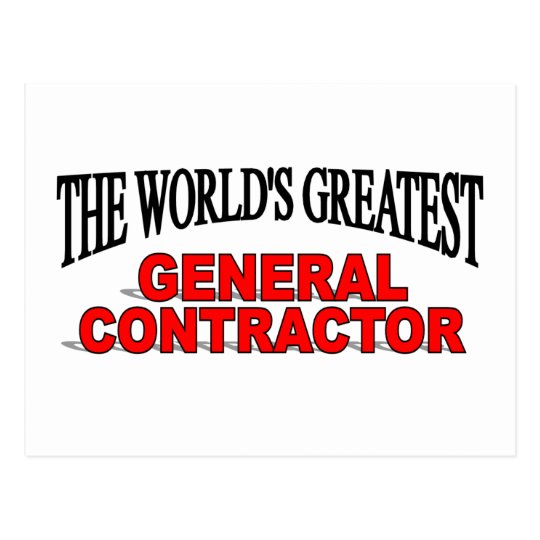The image features two distinct phrases on a plain white background. At the top, "THE WORLD'S GREATEST" is displayed in a black, capitalized serif font that has a distinctive circus-like style, reminiscent of the fonts seen on old circus tents and trucks. This phrase arches gently in a concave shape, hugging an imaginary circle. Below it, centered, is "GENERAL CONTRACTOR," written in a bright red, blocky sans serif font with a black outline. These words are thicker and are accentuated by a gray drop shadow that falls behind and to the left of the letters, adding depth to the image. The stark contrast between the black and red fonts against the white background makes the text stand out prominently.